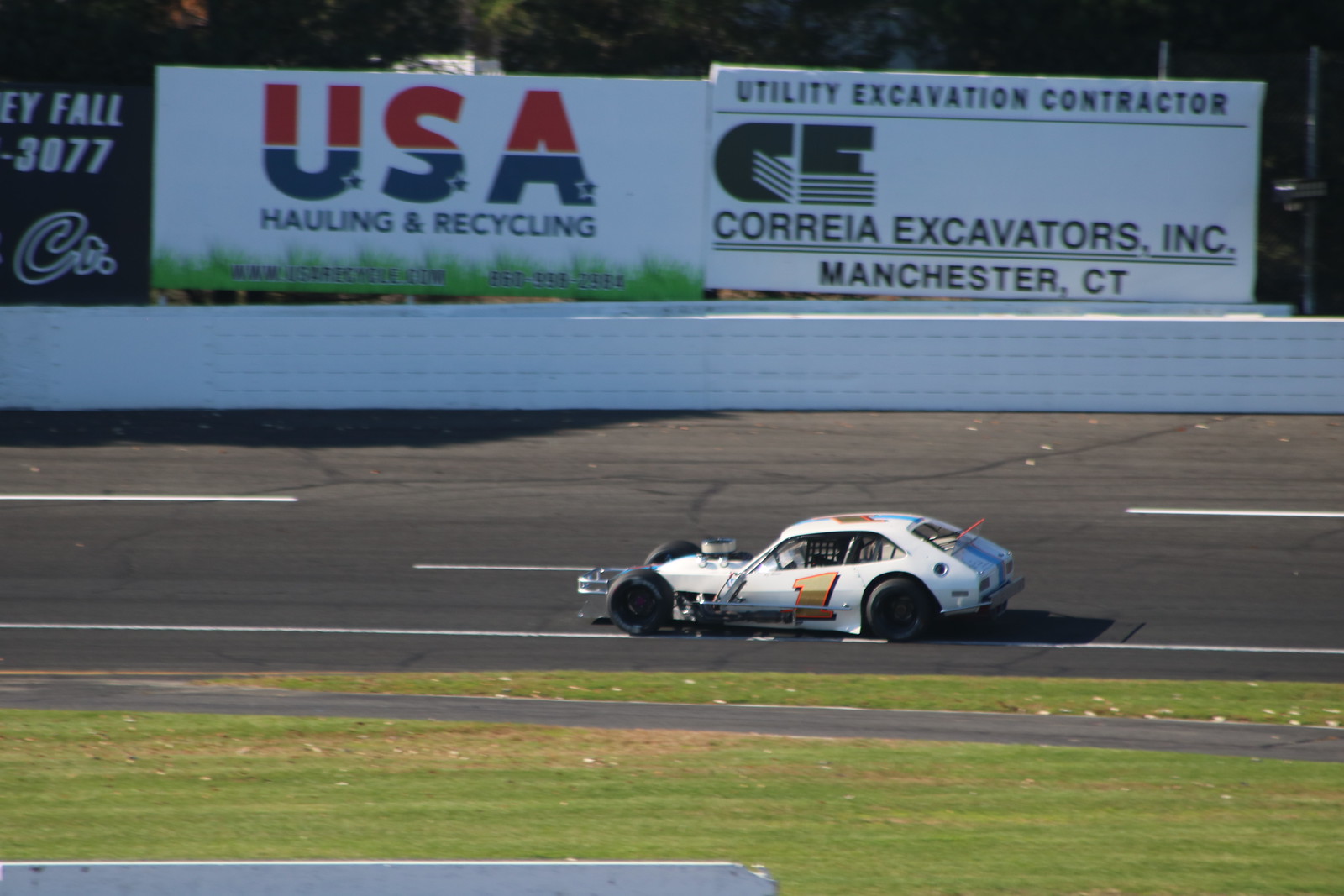This image captures a high-speed moment on a racetrack featuring a souped-up white dragster-like race car. The car, which has large black tires that protrude above its small front end, is emblazoned with a bold gold-colored number one, outlined in orange, on its side. Inside, a racing net is visible, emphasizing its purpose-built design. The car zooms past on a black track, surrounded by a verdant stretch of green grass in the center of the track. A white barrier wall separates the track from the background, where several advertising billboards are visible. Prominent among them, on the right, is a sign for "Utility Excavation Contractor, C.E. Correa Excavators, Inc., Manchester, Connecticut," while to the left, another billboard reads "USA Hauling and Recycling" in red and blue letters. The well-maintained track and detailed advertisements suggest a professional racing event, possibly taking place in Connecticut.